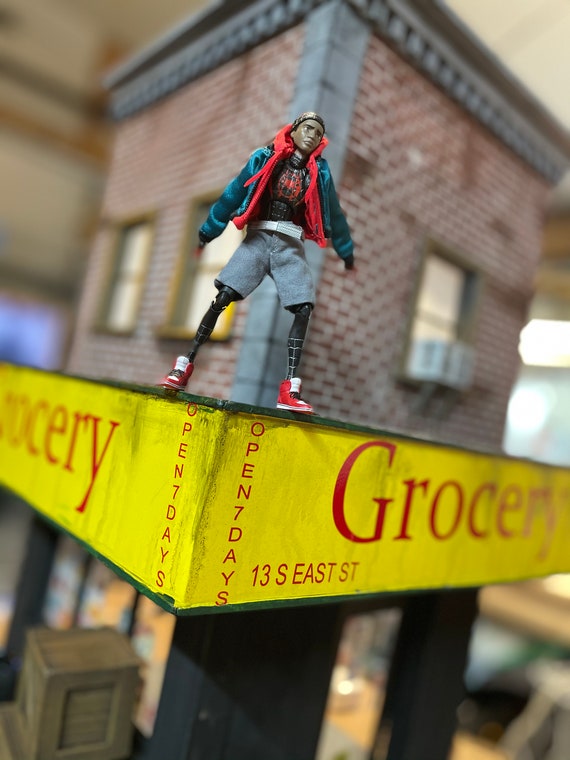The image depicts a realistic miniature playset featuring an action figure of Spider-Man dressed in casual street clothes. The meticulously detailed brick building is two stories tall with a flat roof and several windows, one of which has an air conditioning unit. A yellow sign attached between the upper and lower floors reads "Grocery" in red letters, followed by "Open 7 Days" and "13th of Southeast Street." Spider-Man stands on top of this sign. He sports skinny black legs, red and white sneakers, gray shorts, a black Spider-Man suit under his clothes, a red hoodie, a blue jacket, and a black beanie. The setting is enhanced with realistic touches, including dirt marks on the sign and a blurred red brick background.